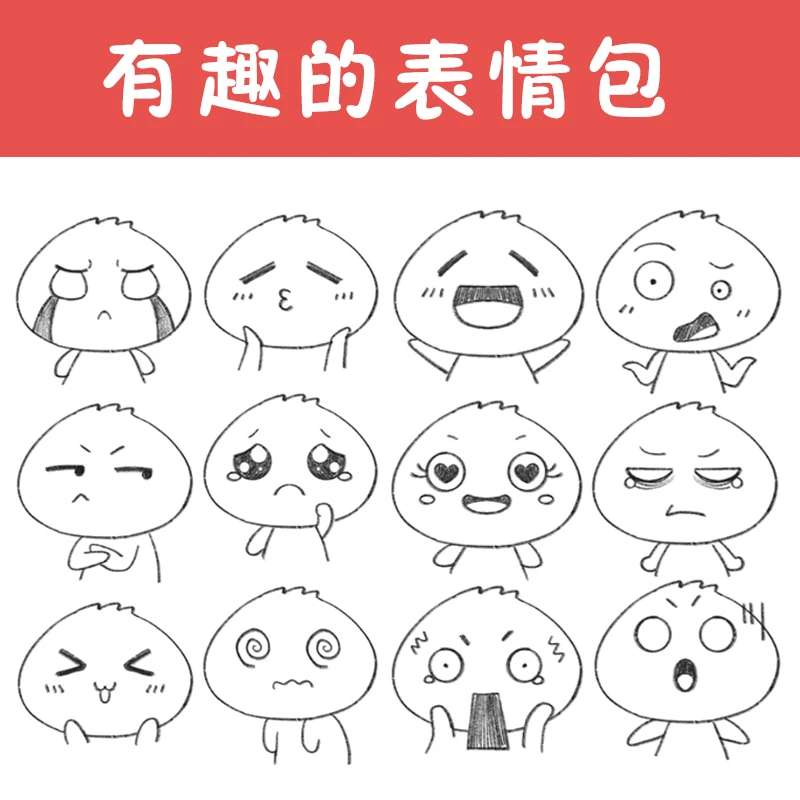The image is a large square poster titled "Emotions," featuring a series of simple line drawings in the shape of round, chicken-like characters that depict various facial expressions. These characters are arranged in three rows on a white background. At the top of the poster, there is a prominent red band containing white Chinese characters. Each character has a round head with three spikes of hair, and their expressive faces comprise circles for eyes and lines for mouths. The emotions portrayed include crying, kissing, happiness, confusion with raised shoulders, anger, shock, heart eyes, sadness, tiredness, tongue out, arms crossed with side eye, and a combination of being upset and crying.